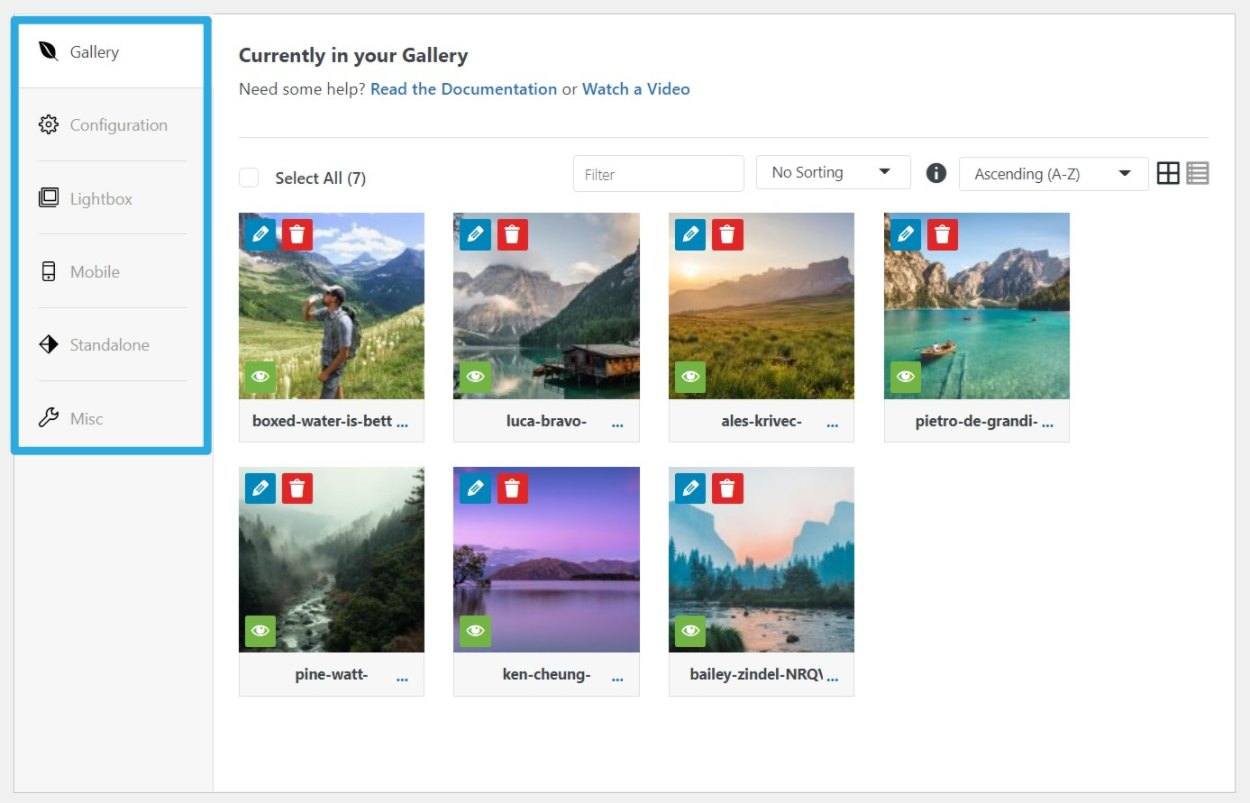**Caption:**

The interface displays a side menu on the left, enclosed within a blue rectangular outline. This menu is structured as a list, featuring the following options each with an icon on the left:

1. **Color** - Represented by a black leaf icon.
2. **Configuration** - Indicated by a black gear lever icon.
3. **Light Box** - Marked by a box icon.
4. **Mobile** - Depicted by a cell phone icon.
5. **Stand Alone** - Illustrated with a diamond icon.
6. **Misc** - Symbolized by an orange gear icon.

At the top of the main page, a text reads "Currently in your gallery" in black, followed by two options in blue text: "Need some help? Read the documentation or watch the video."

At the bottom, there's a "See All" section followed by a checkbox, indicating seven items are visible.

In the toolbar, there are several controls:
- **Filter** dropdown menu.
- **Settings** dropdown.
- Sorting option "Ascending A to Z."
- **View** options: Grid view and List view, located on the far right.

On the main page, the top left corner displays seven pictures, each overlaid with three colorful patterns: a blue right pattern, a red direct pattern, and a green eye pattern on the bottom left.

The images feature various descriptions and names:
1. **Picture 1:** "Boxed Water is Better"
2. **Picture 2:** "Luca Bravo"
3. **Picture 3:** "Alice Krivak"
4. **Picture 4:** "Pietro De Grandi"
5. **Picture 5:** "Pine Water"
6. **Picture 6:** "Ken Chong"
7. **Picture 7:** "Bailey Zindel"

These images showcase landscapes of mountains and lakes, alongside some featuring dams.